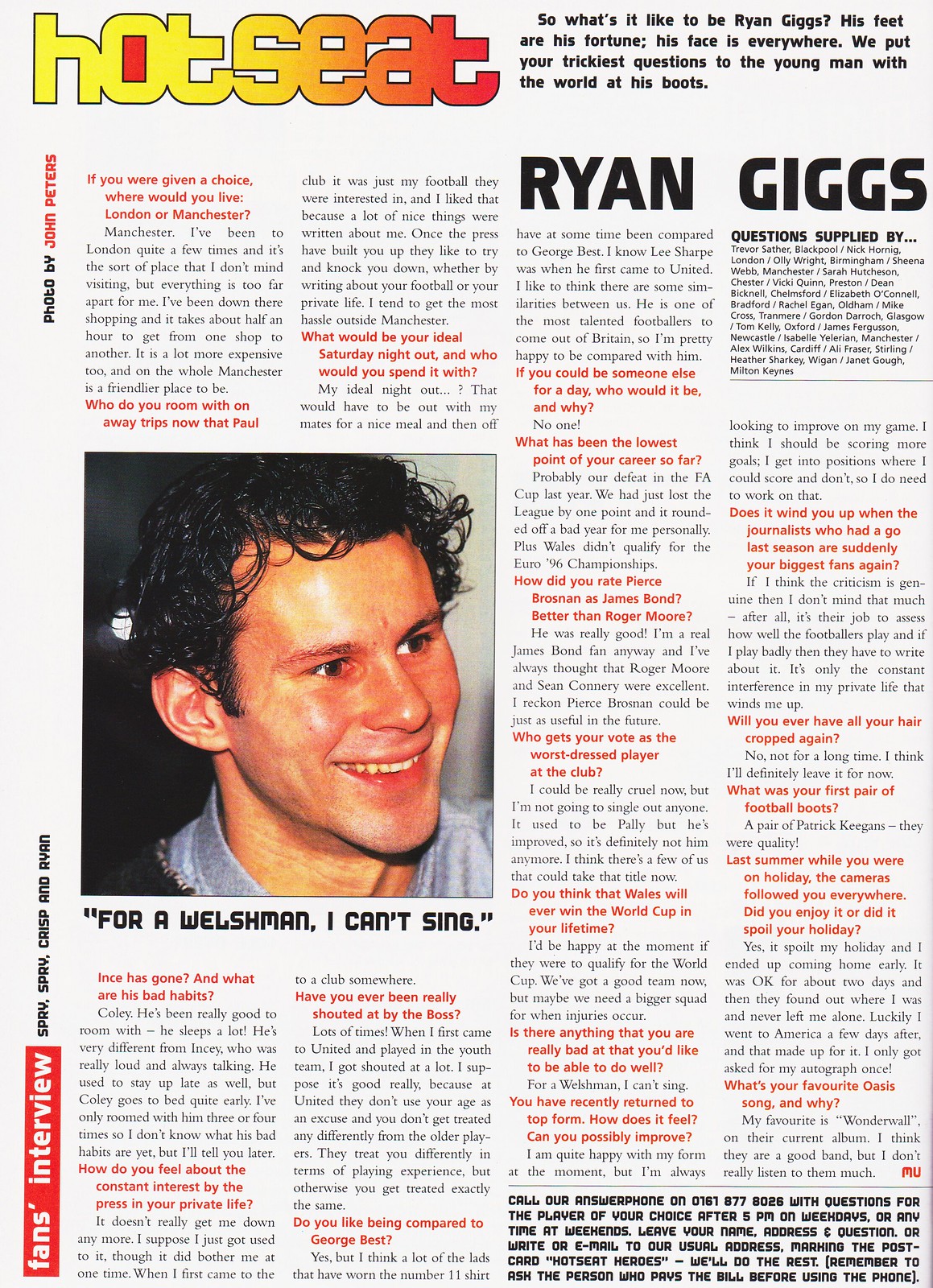The image portrays a page from a magazine article, chiefly focused on Ryan Giggs. In the upper left corner, there's a distinctive gradient logo that transitions from yellow to orange to red, reading "HOTSEAT" in bold capital letters. Right beside it, in bold text, appears the name "Ryan Giggs." 

The image prominently features a headshot of Ryan Giggs on the left side, occupying about a third of the page's height, and his body faces forward while he looks towards the 4:30 position with a smile. He appears young, possibly in his early 20s, with medium-length curly hair. Underneath his photograph, there's a quote attributed to him: "For a Welshman, I can't sing."

In addition to the visual elements, the article includes several paragraphs of text, indicating it's not the article's opening page since it starts mid-sentence. A notable line reads, "So what's it like to be Ryan Giggs? His feet are his fortune. His face is everywhere. We put your trickiest questions to the young man with the world at his boots." The text suggests an interview format where one question reads, "If you were given a choice, where would you live? London or Manchester?" to which the answer noted is "Manchester."